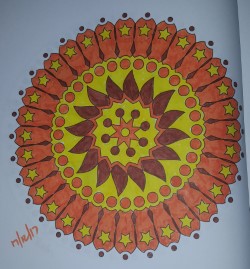The image depicts a small, intricately designed blue square featuring an ornate mandala pattern. At the heart of the mandala lies a yellow center adorned with maroon accents, surrounded by numerous red dots and flame-shaped elements extending outward. Encircling this central motif are shapes reminiscent of traffic parking meter tops, each with a pointed tip and a red exterior with yellow centers. The detailed craftsmanship and vibrant colors create a mesmerizing visual effect. Adding a personal touch, a signature is visible on the left-hand side of the image.